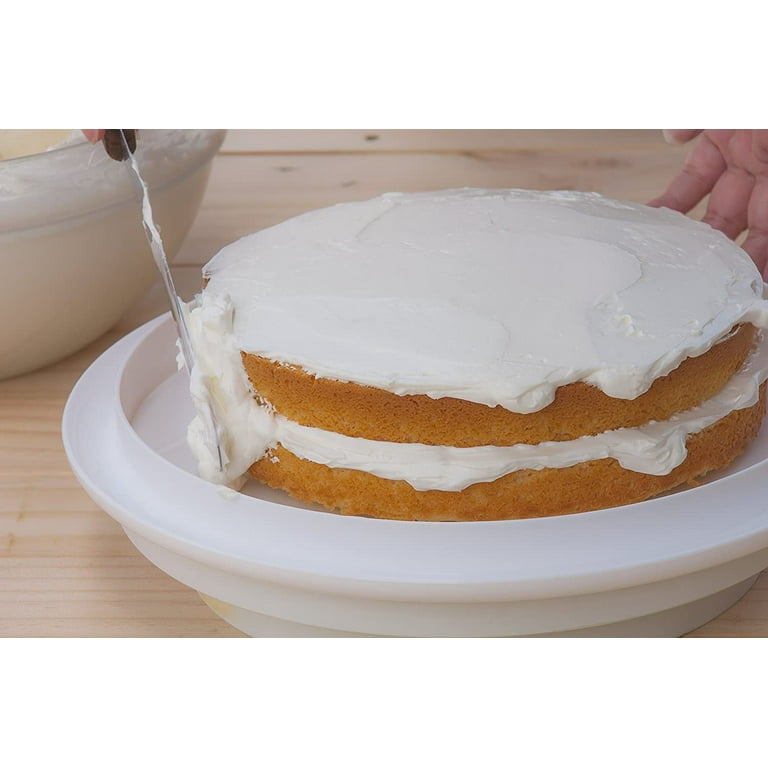The image captures a close-up of a simple yet elegant cake-decorating process. Centered on a light brown wooden table, the scene features a two-layer vanilla cake with a layer of white frosting in the middle. The cake is perched on a white dish with a tall rim, designed specifically for presenting cakes. The cake appears rich and moist, its yellow-brown sponge contrasting subtly with the white buttercream frosting being meticulously applied. A person's hand, positioned in the top right corner, is using a thin metal spatula to spread the frosting evenly around the sides of the cake. The setting is likely a kitchen, indicated by a partially visible white mixing bowl in the upper left corner. The focus is clearly on the careful icing technique, capturing a moment of delicate culinary craftsmanship.